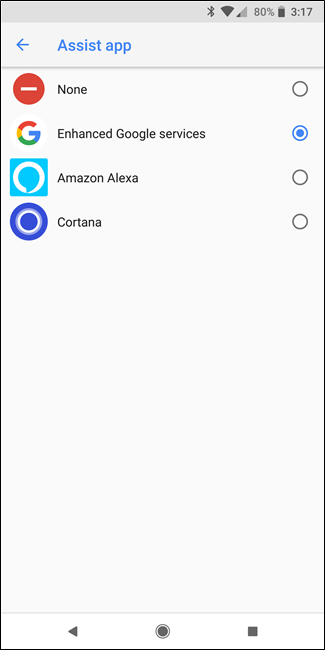This image depicts a smartphone screen displaying various features and icons. The battery indicator shows a charge level of 80%. Bluetooth connectivity is active. The interface includes an app icon labeled "Tom" with a value of 317, as well as an "Assist" app. There is a left-pointing arrow at the bottom of the screen. 

Additionally, the screen shows three unshaded radio dial buttons, each corresponding to different services: enhanced Google services, Amazon Alexa, and Cortana. 

At the bottom of the screen, there are navigation icons including an arrow pointing left, a circle, and a square.